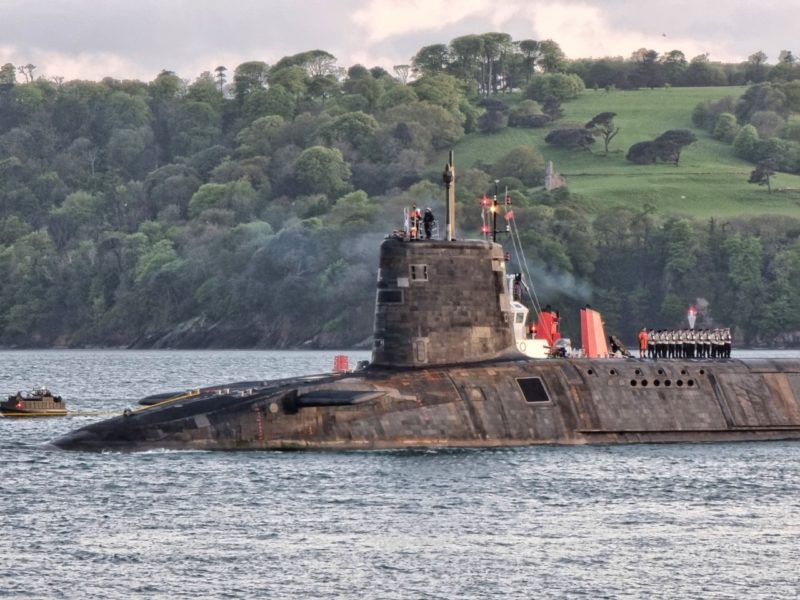In the foreground of the image, a weathered, dark brown, and almost rusty submarine floats serenely in calm, gray-toned water. The top part of the submarine is prominently above the surface, featuring a metallic tower towards the front. On the submarine's deck, a group of sailors is lined up in formation, most of them wearing gray tops and black trousers, with one distinctively in red. Among them, two men stand higher on the tower. To the left, another boat, likely modern, is tethered to the submarine, suggesting it transported the sailors. In the background, a landscape of lush green-leafed trees blankets the distant hills, with a field of well-maintained grass resembling a golf course clearing on the right. The sky is a moody mix of gray and white clouds, casting a muted light over the scene.